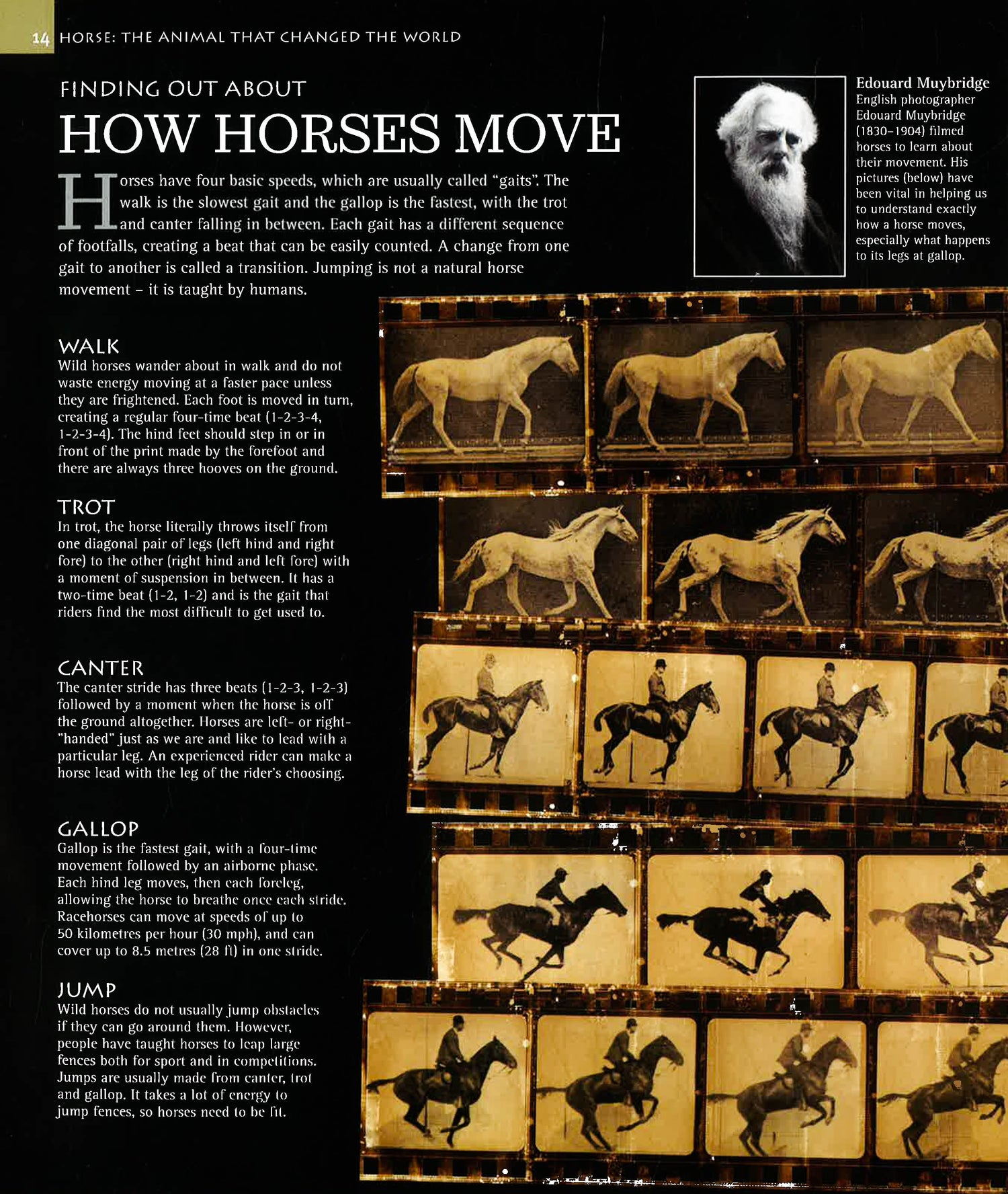The image is a detailed poster with a black background and white text primarily positioned on the left side. The text at the top reads, "Horse, the animal that changed the world" and "Finding out about how horses move." Below this headline, there are five to six paragraphs elaborating on the various movements of horses. The top right corner features a black and white photo of Edward Muybridge, accompanied by a textual description of him, including his significance in capturing the movement of horses. The text identifies Muybridge as an English photographer (1830-1904) who significantly contributed to our understanding of horse locomotion.

The right half of the poster displays around 15 to 20 vintage-style photographs of horses arranged in five rows. The top two rows show white horses without riders in various stages of movement. The remaining three rows depict black horses being ridden by jockeys, also in different strides. Each image is labeled with the specific movement it represents, such as walk, trot, canter, gallop, and jump. The captions detail the sequence of footfalls and explain how each gait is unique. The text on the left side also mentions that horses have four basic speeds, known as gaits—walk, trot, canter, and gallop—with jumping being an unnatural movement taught by humans.